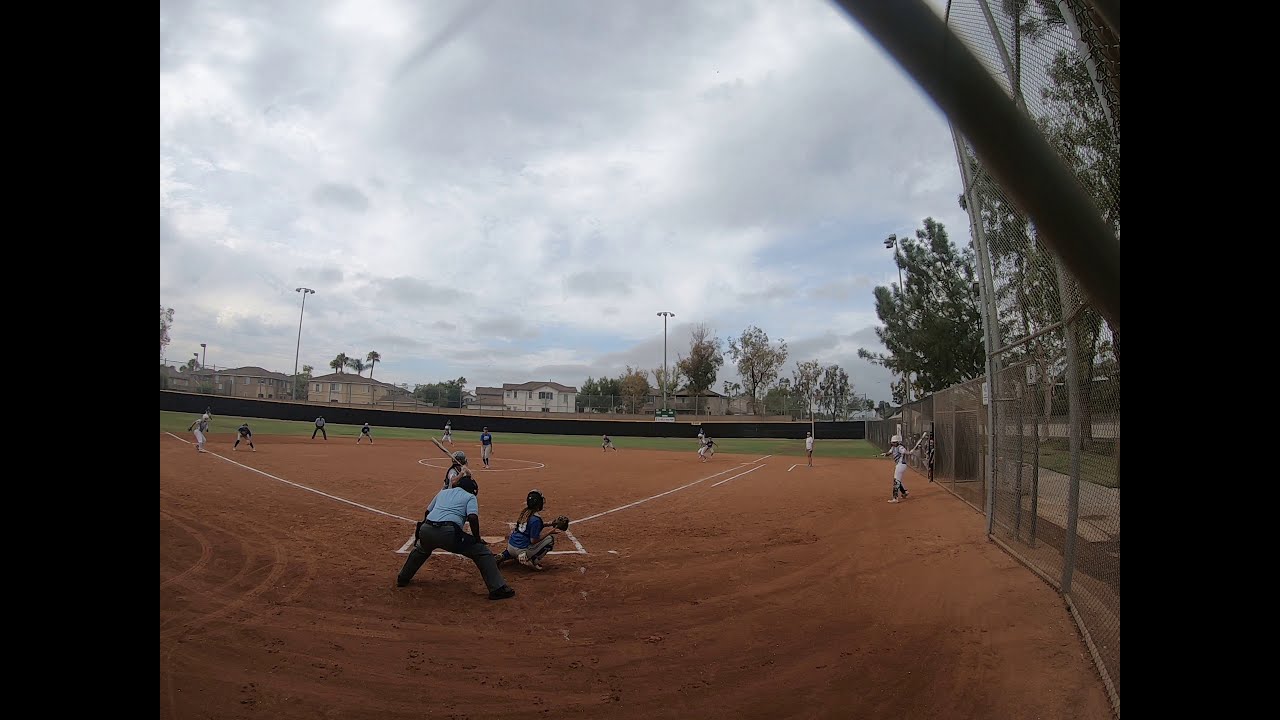This photograph captures a baseball game from behind home plate, providing a comprehensive view of the field and its surroundings. The umpire, in a light blue shirt and black pants, is crouched behind the catcher, who is wearing a blue jersey with either the number zero or eight and gray pants, and is poised with their mitt, ready to receive a pitch. The batter, partially obstructed by the umpire, holds the bat up, prepared to swing. 

The players are positioned throughout the sand infield and grassy outfield, with the pitcher clearly visible on the mound and various fielders in place. A brown wall marks the boundary of the field, beyond which lies a residential neighborhood featuring tan and white houses interspersed with green trees. The sky overhead is mostly cloudy with only a small patch of blue peeking through, casting a diffused light over the scene. The setting is adorned with a metal fence encircling the diamond, and a sidewalk runs just outside the park, emphasizing the suburban backdrop.